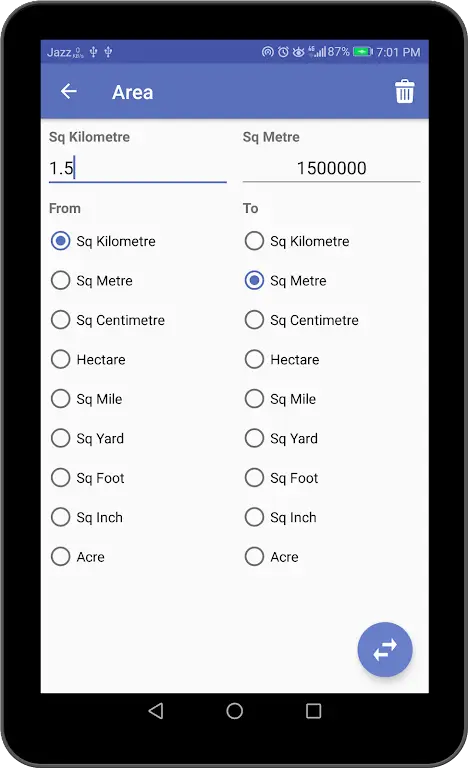The image depicts a compact cell phone with a screen surrounded by a black bezel. The phone features the traditional navigation buttons—a triangle, a circle, and a square—located on the black bezel below the screen rather than integrated into the display. 

The top of the screen displays a dark blue status bar. "Jazz" is shown on the left side of the status bar, indicating the network provider or some related information. To the right of this, there are two USB connection symbols. On the far right, there are various icons: a hotspot activation icon, an alarm icon, an eyeball icon (the purpose of which is unclear), full carrier signal bars, a battery icon indicating 87% charge, and the current time, 7:01 PM.

Below the status bar, there is a medium blue bar, which is approximately twice the thickness of the status bar. In this blue bar, there is white text with the word "Area" followed by a left-pointing arrow on the left side, and a white trash can icon on the right side.

The main part of the screen has a white background. On the left, "SQ Kilometer" is displayed, followed by the value "1.5" with a cursor positioned right after it. Below that, the word "From" is shown, indicating the selection of square kilometers. On the right side, "SQ Metre" is listed, alongside the value "1,500,000," suggesting a conversion from 1.5 square kilometers to 1,500,000 square meters.

Additionally, a section shows options to convert area units. On both sides of the screen, the available units for conversion are displayed: square kilometer (SQ Kilometer), square meter (SQ Metre), square centimeter (SQ Centimeter), hectare, square mile (SQ Mile), square yard (SQ Yard), square foot (SQ Foot), square inch (SQ Inch), and acre.

In the bottom right corner of the screen, there is a blue circle featuring a white right-pointing arrow, and below this, a smaller white left-pointing arrow.

The overall interface suggests that the image captures a phone in the process of converting area measurements between different units.